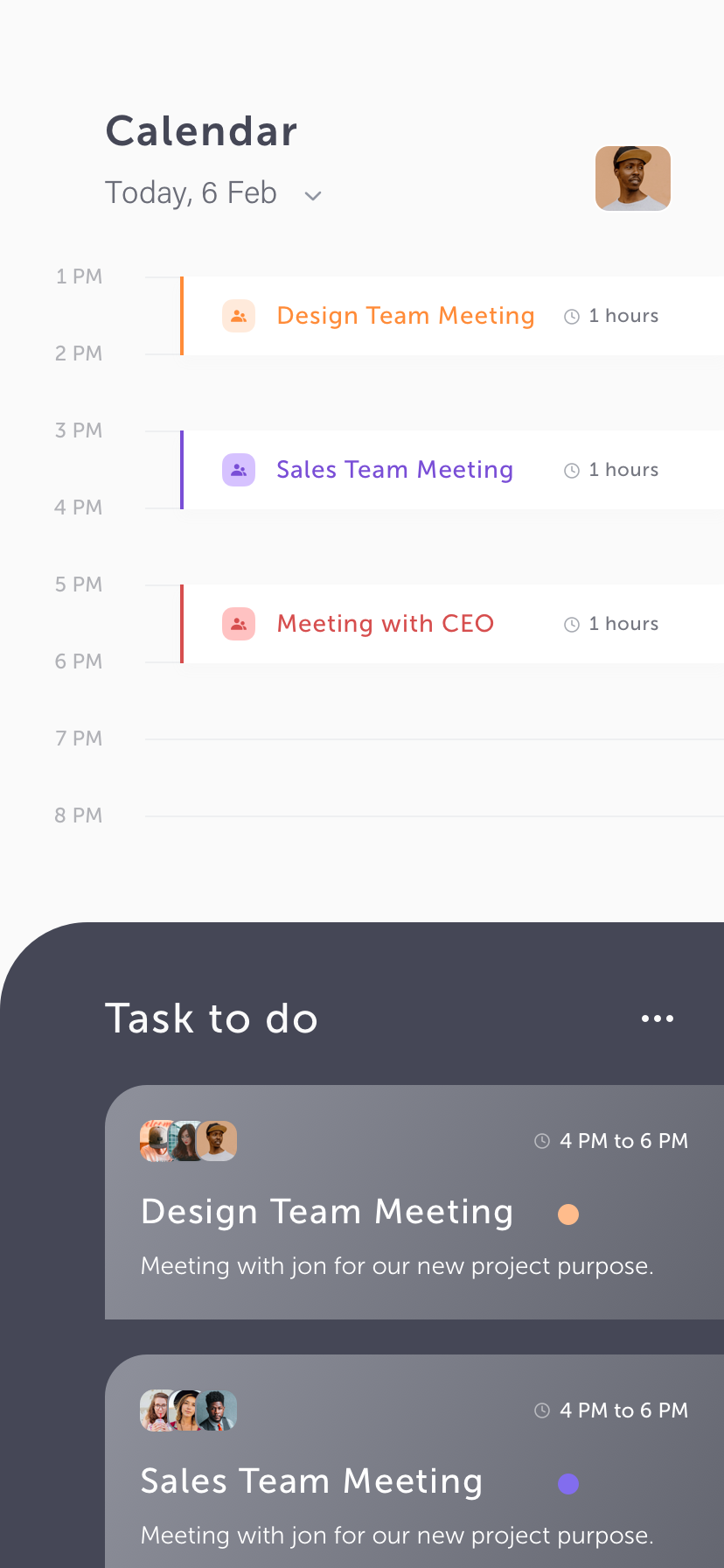A detailed close-up of a desktop calendar for February 6th is displayed. The header reads "Calendar" with the date prominently marked as "Today, 6th February." The timeline spans horizontally from 1 PM to 8 PM. Three meetings are scheduled for the day:

1. **Design Team Meeting** from 1 PM to 2 PM, highlighted in orange.
2. **Sales Team Meeting** from 3 PM to 4 PM, marked in purple.
3. **Meeting with CEO** from 5 PM to 6 PM, indicated in red.

Below the scheduled events is a list of tasks detailing the same meetings, accompanied by profile pictures of the respective participants for each meeting. The image provides an organized snapshot of a busy professional day.